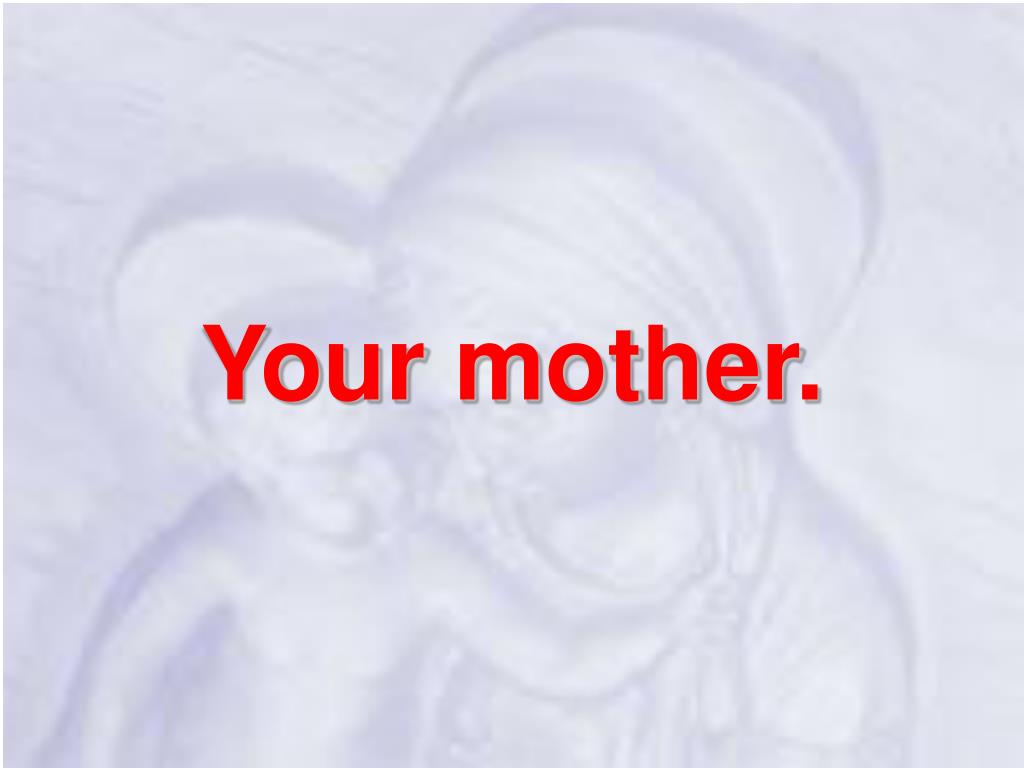The digital image is a nearly square rectangle with a light gray and white background, featuring varying hues of gray that subtly transition into a lavender tone. In the center of this backdrop, the phrase "your mother." is prominently displayed in large, red letters, casting a slight shadow to the right. Embedded within the gradient background is a faint, yet discernible, digital image resembling the Virgin Mary holding baby Jesus. Both figures have halos above their heads. The baby is depicted reaching out to tug either at the Virgin Mary's headscarf or hair. The figures, visible from the top of the Virgin Mary's head to just below her shoulders and down to the baby's waist, appear almost three-dimensional, akin to an artistic rendition on pressed paper. This effect creates the illusion of shadows forming the lines, adding depth to the spiritual imagery in this religious-themed artwork.